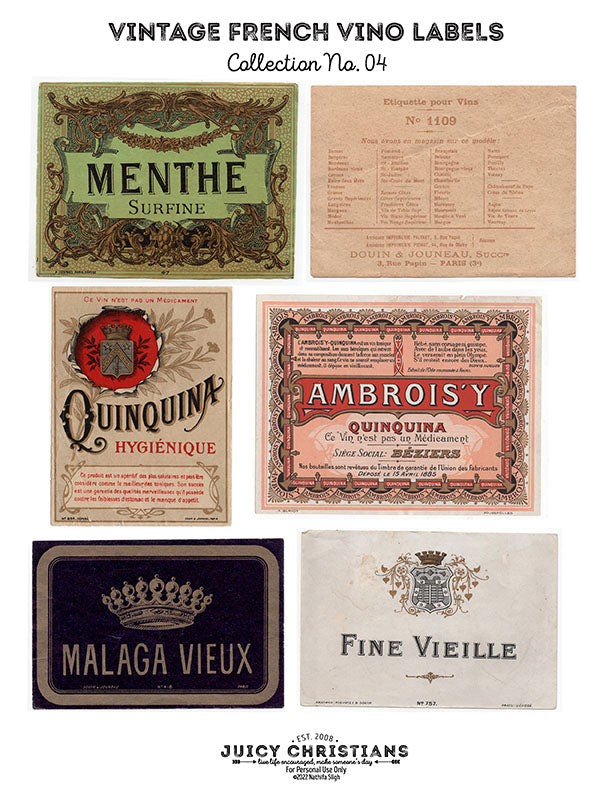This image features a meticulously arranged poster titled "Vintage French Vino Labels," showcasing a collection of six distinct vintage French wine labels. The title "Collection Number 4" is emblazoned in black cursive text at the top of the poster. 

In the top left corner, a label with the title "Menthe" is set within an ornate decorative frame with a refined green and brown color scheme. Adjacent in the top right, a label resembling a descriptive document or catalog page features a beige background with the number 1109 prominently visible, mentioning "Dwan des Jeunes Sucs" and an address in Paris.

Moving to the middle left, a vibrant label marked "Quinquina" stands out with large red letters and a crest above it. To the right of it is a red and light brown themed label with the term "Ambrosie" displayed prominently.

At the bottom left, a striking blue label branded "Malaga VO" features a silver crown emblem above its text. Finally, on the bottom right, a light gray label with a small crown is inscribed with the word "Vieille," and a note saying "Juicy Christian" at the bottom. Each label adds to the rich tapestry of vintage French wine culture depicted in this collection.